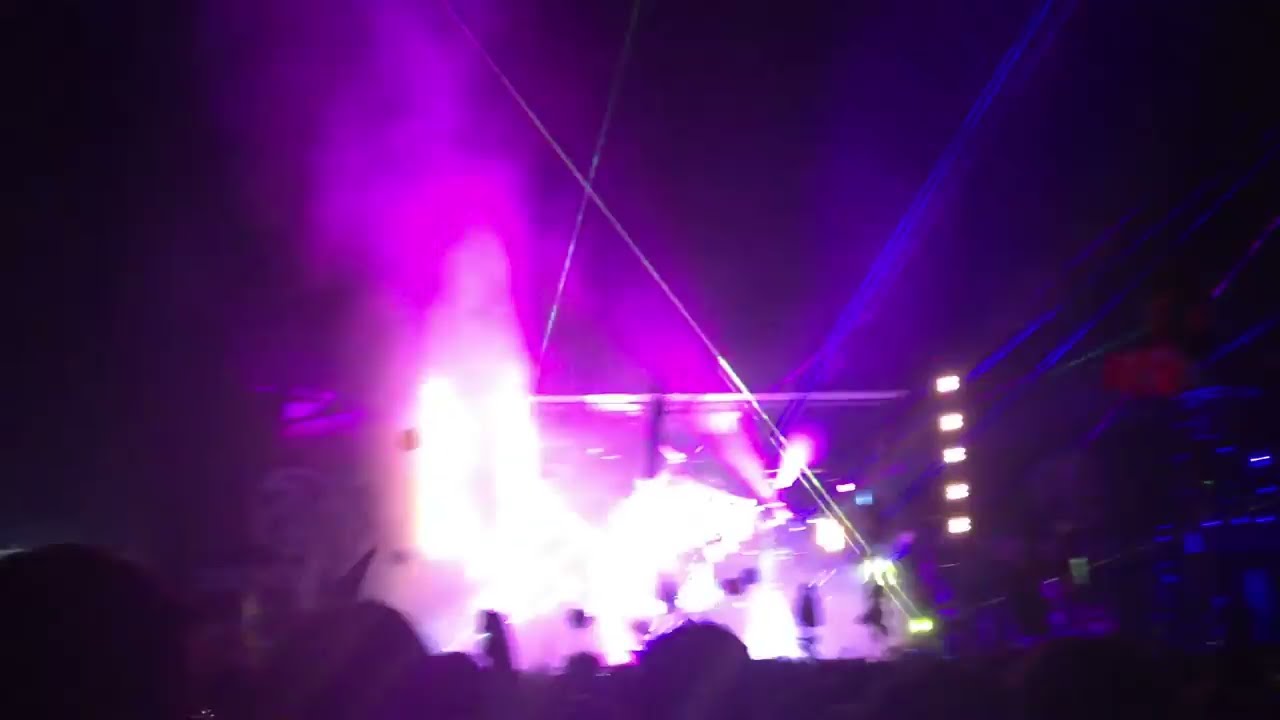The image appears to capture a vibrant, albeit very blurry, moment from a concert. Dominated by purple, pink, and blue hues, the stage is illuminated with a series of five whitish lights ascending a post, and a metal canopy overhead. An explosion of bright lights and vibrant laser beams, resembling lightning bolts of color, emanates from the stage, casting dramatic silhouettes. In the foreground, the dark shapes of audience members can be seen, their heads forming a shadowy outline against the illuminated stage. Despite the blur, you can faintly discern shadows on the stage that might be performers, alongside what seems like a mix of pyrotechnics and laser effects contributing to the intense, energetic atmosphere. In the background, it’s possible to make out more people, potentially in the stands, adding to the impression of a large, exciting concert.